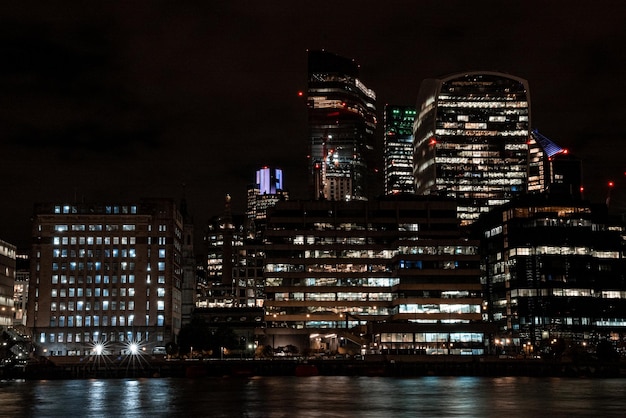This realistic, horizontally-oriented nighttime photograph captures a striking city skyline, possibly reminiscent of New York City. The background is pitch black, accentuating the illuminated cityscape. In the foreground lies a dark body of water, likely a river or bay, which mirrors the lights from the buildings. A row of lower buildings, around 10 to 15 stories high, possibly including a parking garage, fronts the scene. Beyond these, several taller skyscrapers soar into the night, ranging between 20 to 50 stories. The tallest buildings are adorned with bright lighting, including one with a vividly lit blue top and another with red lights for aircraft visibility. Numerous apartment and office windows glow, though not every room is illuminated, creating a mosaic of light against the dark structures. On the left side of the image, a building features a sign, though it's indiscernible due to the darkness. Street lights and other light sources punctuate the scene, making for a well-composed and visually engaging cityscape.